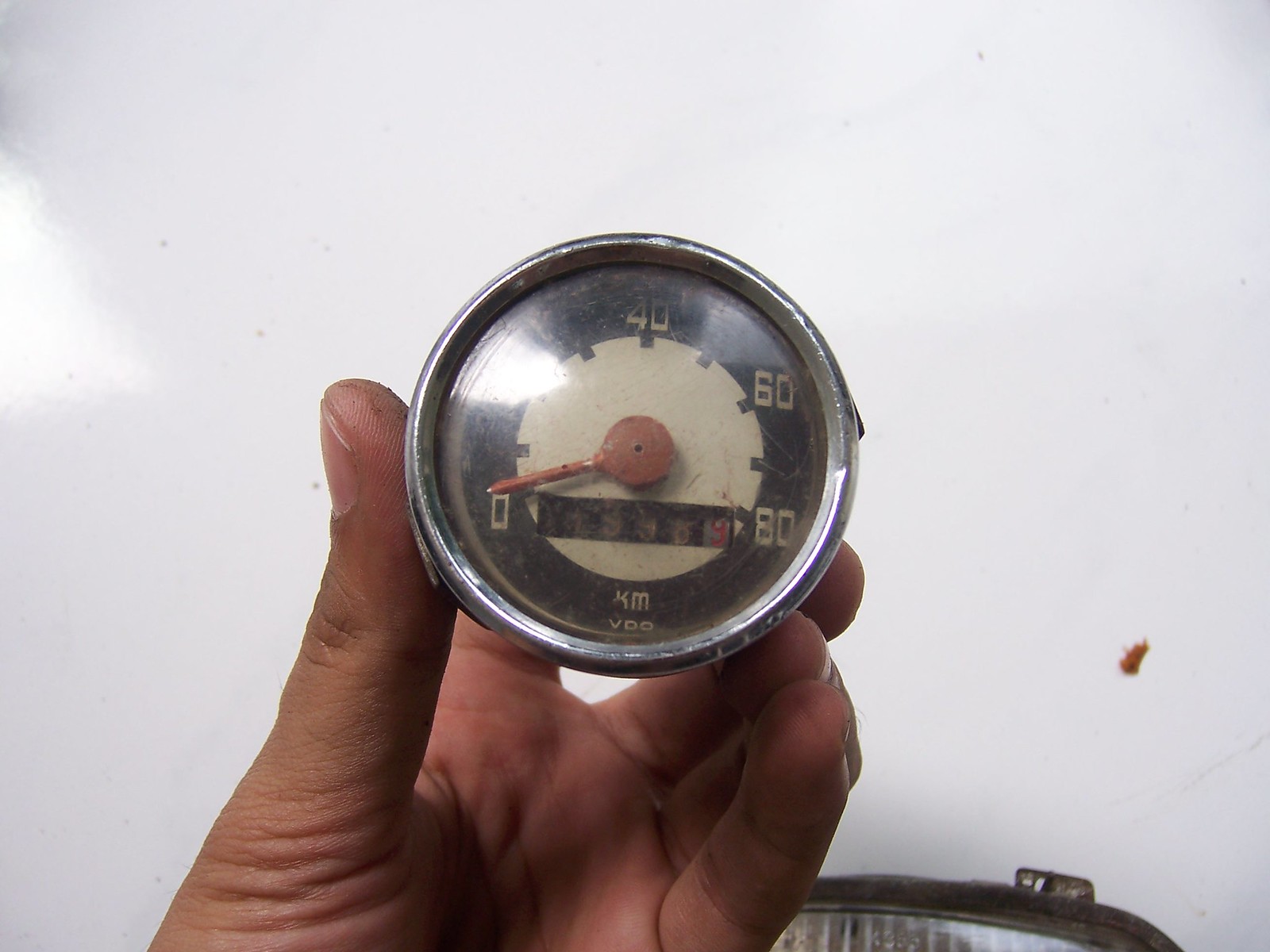A close-up image captures a left hand holding a vintage speedometer/odometer against a stark white wall. The hand, slightly dirty around the thumb, grasps the gauge delicately between the thumb and middle and ring fingers. The speedometer itself features a metal rim that protrudes slightly from its surface, indicating wear and age. The face of the gauge, encased in a clear but somewhat grimy plastic cover, displays a large black circle with a smaller white circle inside. Numbers ranging from 0 to 80 in yellow font encircle the black background in increments of 20. A red needle points just above the zero mark. A bright white spot, possibly from a light source, is visible on the top left of the speedometer's face, while a peculiar reddish speck appears in the bottom right quadrant of the image. To the left of the gauge, a rusted silver metal object, seemingly attached to the wall, adds to the overall vintage ambiance of the photograph.